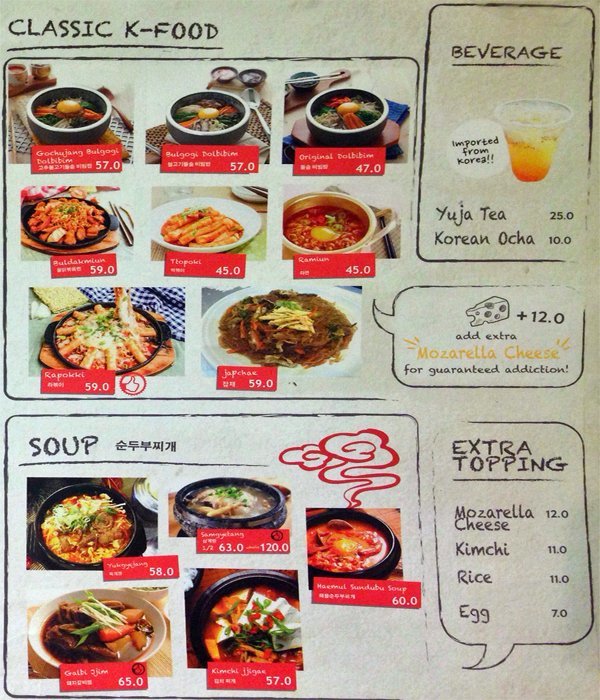This image depicts a Korean restaurant menu, characterized by a blend of printed and handwritten elements on a white-grayish background. The menu is divided into two main sections: "Classic K-Food" at the top and "Soup" at the bottom. The "Classic K-Food" section features eight dishes organized into three rows: three dishes in the first row, three in the second, and two in the third. Each dish includes a photo, and beneath each photo, there is a red box with white lettering detailing the name and price of the dish.

On the right-hand side of the menu, there are three distinct sections. At the top is the beverage section, housed within a black box that includes an image of a red and orange drink, likely tea, with options such as yuja tea and Korean oka along with their prices. Below this is a box highlighting additional toppings, including an option to add extra mozzarella cheese for an additional cost and the enticing description "mozzarella cheese for guaranteed addiction." The third box at the bottom right focuses on extra toppings, listing options like mozzarella cheese, kimchi, rice, and egg, each with their respective prices.

The "Soup" section at the bottom of the menu is outlined in black and features five different soups, arranged in two rows: three in the top row and two in the bottom row. Similar to the dishes above, each soup is displayed with a photo and accompanied by a red box that includes the name and price. The overall layout is visually organized yet retains a casual, handwritten feel, making it inviting and easy to navigate.